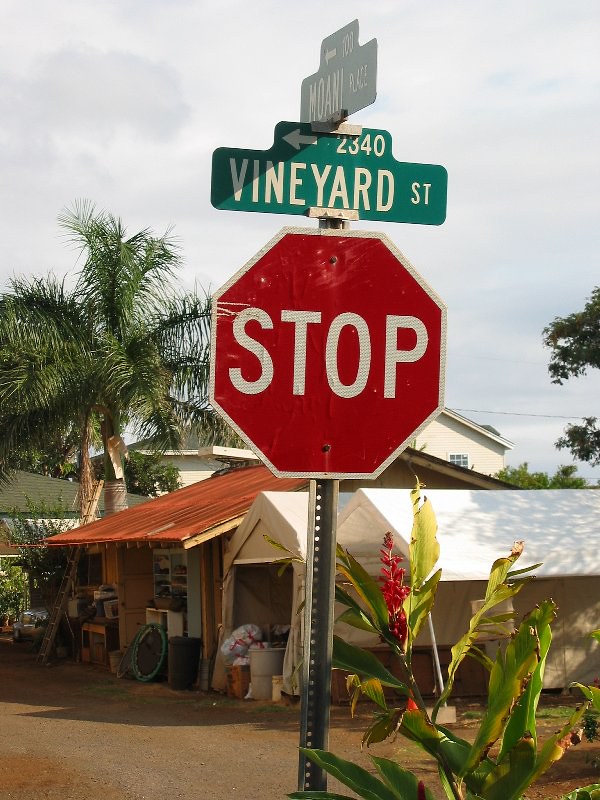In the foreground, a classic red stop sign with bold white lettering commands attention. Just above it, a green street sign indicates "Vineyard Street" with an arrow pointing to the left, accompanied by the number "2340." Facing the opposite direction, another green street sign can be seen. The background is dominated by lush green palm trees with sturdy brown trunks.

Adjacent to these tropical trees is a building featuring a red porch, with two white tents positioned next to it. Initially appearing to shelter a person bending over, it becomes evident that beneath the middle tent are trash bags. Nearby, a gray trash can and a black trash can are placed side by side. To the left of these bins, a blue ring with a black center is discernible.

Also to the left, a large silver ladder extends upward into one of the palm trees. In the backdrop stands a stately three-story house, resplendent in white with a contrasting gray roof. Completing the scene is a vibrant green leaf plant situated in front beside the stop sign.